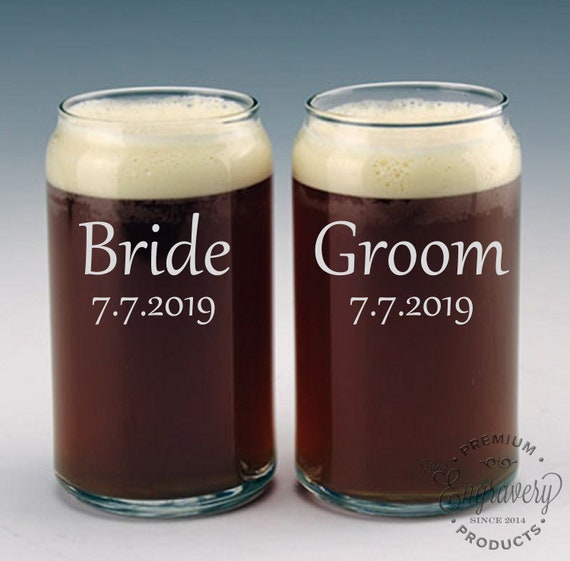This professionally staged, full-color product photograph features two matching clear glass cups, each designed to resemble an open-top Lumum soda or beer can. They are filled with a dark brown liquid topped with white foam. The cups are side-by-side, with the left cup labeled "Bride 7-7-2019" and the right cup labeled "Groom 7-7-2019," both in white text. The image, predominantly square in format, has a gradient background transitioning from dark gray at the top to light gray at the bottom, enhancing the product's visibility. In the bottom right corner, a circular watermark reads "Premium Products by Engravery Since 2014," attesting to the brand's quality. This style of meticulous, realistic product photography is ideal for commercial listings such as online shops and catalogs.